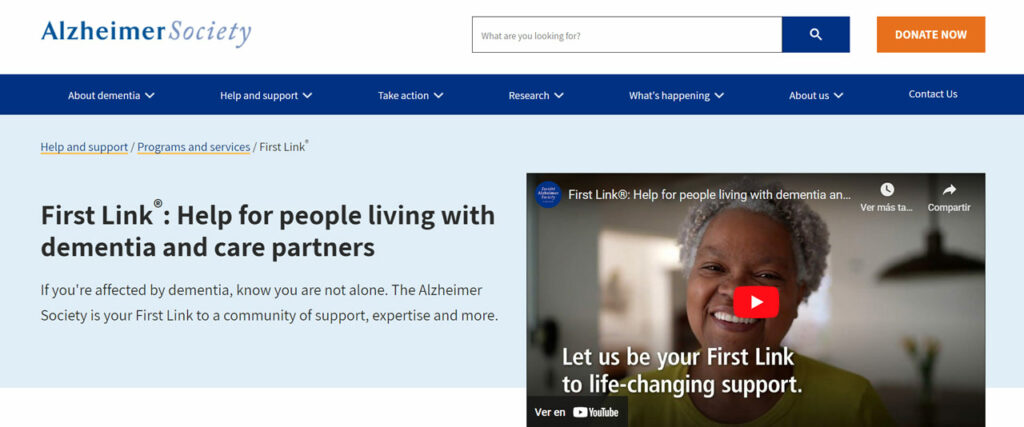In the top left-hand corner of the web page, a blue logo reads "Texas Alzheimer's Society." To the right of this logo is a search bar with the placeholder text, "What are you looking for?" Next to the search bar is a blue button featuring a white magnifying glass, and beside it, an orange button with white text that reads, "Donate Now." Below these elements is a horizontal blue navigation bar with several drop-down menus labeled: "About Dementia," "Help and Support," "Take Action," "Research," "What's Happening," "About Us," and "Contact Us." All categories, except "Contact Us," feature arrows indicating additional menu options.

Continuing down, a light blue box displays the following text: "Help and Support / Programs and Services / First Link." Below this, it states, "First Link: Help for people living with dementia and care partners. If you're affected by dementia, know you're not alone. The Alzheimer's Society is your first link to a community of support and expertise."

To the right of this section, an embedded video is titled "First Link: Help for people living with dementia and..." The video thumbnail features an elderly Black woman with gray curly hair, dressed in a yellow shirt, smiling. Overlaid on the thumbnail is a white YouTube play icon. In the bottom left corner of the thumbnail, some text is partially visible, showing "ver" and the YouTube logo, while in the top right, partial text reads "ver a..." The video appears to be cut off, indicating it may need adjustment for full visibility.

Below the video thumbnail, white text reads, "Let us be your first link to life-changing support." 

This detailed description succinctly encapsulates the web page's layout and content, focusing on key elements that provide navigation and support for those affected by dementia.